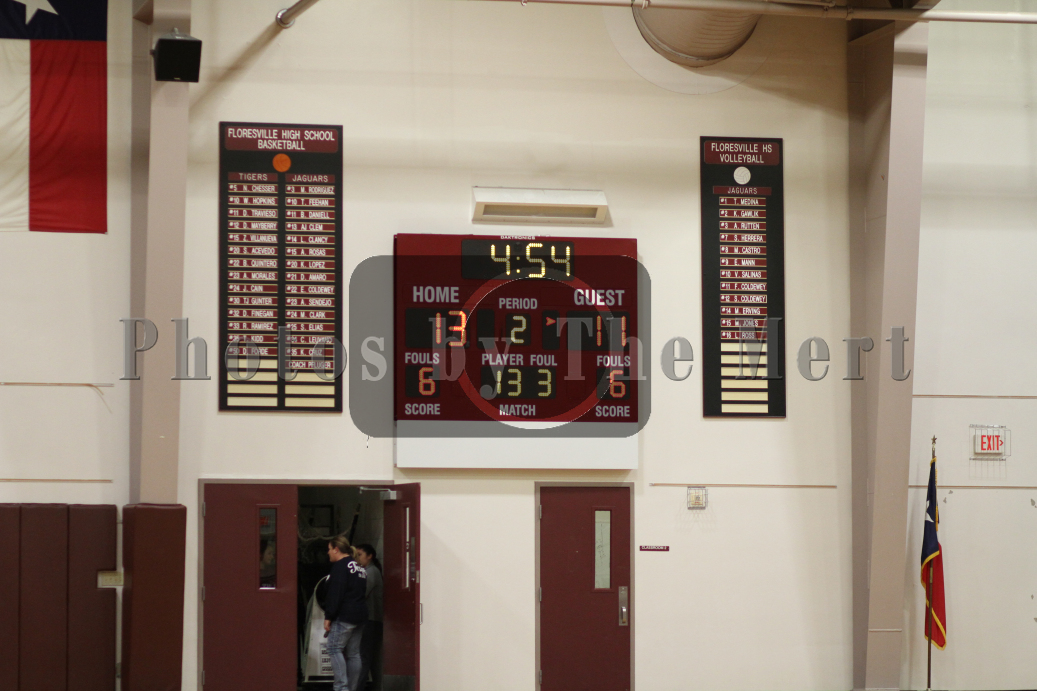The photo captures the interior of a large gymnasium, prominently featuring a wall adorned with various elements. To the left, a Texas flag hangs from the ceiling, featuring a dark blue rectangle with a white star above white and red rectangles. Central to the image is an electronic scoreboard displaying the ongoing sports event's details. The scoreboard, set against a tall, plain white wall interspersed with gray pillars, shows "454" in yellow at the top, indicating the remaining time. Below this, the home team leads with 13 points in red lighting, whereas the guest team has 11 points in red lighting, with both teams having accumulated 6 fouls each. The display reflects it’s the second period of the game. Beneath the scoreboard are two red doors, in one of which, two people are visible. Flanked to the left of the scoreboard are large banners highlighting awards and records for Floresville High School basketball. Below these banners are brown cushions padding the base of the wall. The image also includes an exit sign and more red doors at the bottom of the shot, further emphasizing the functional and scholastic nature of the space.